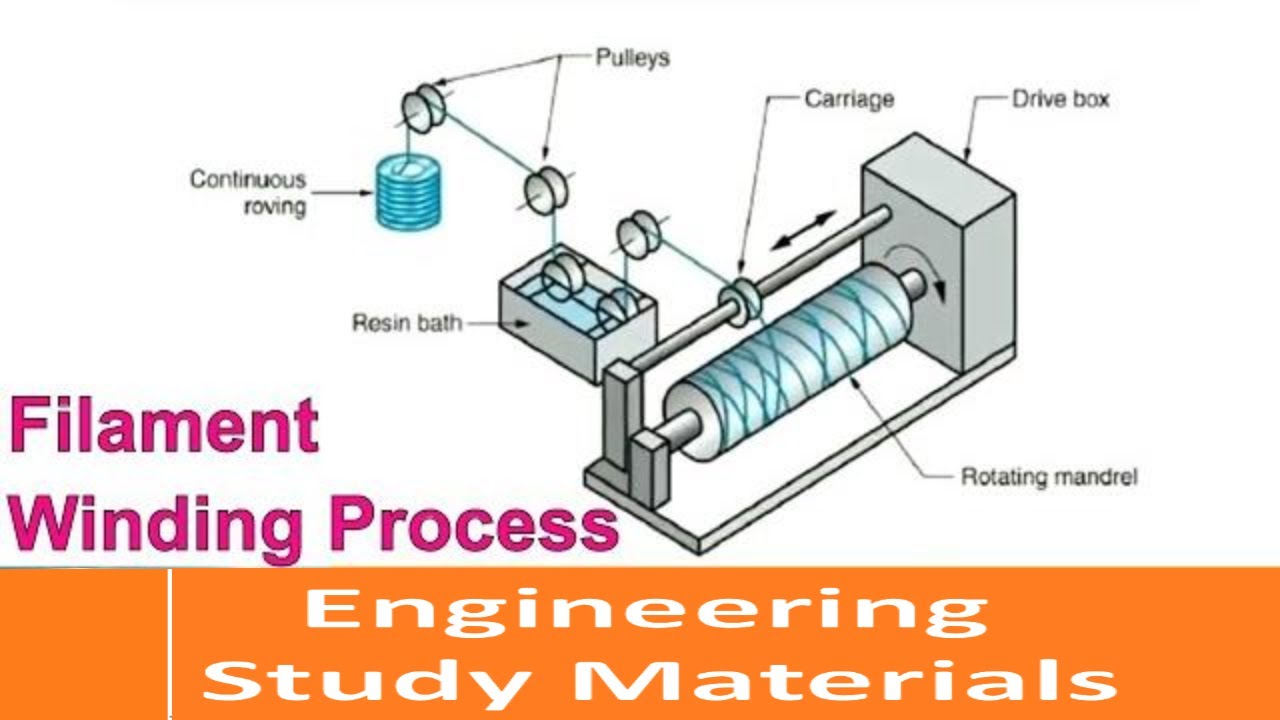The diagram illustrates the filament winding process, prominently labeled in purple bold text on the left and tagged as "Engineering Study Materials" in white text on an orange border at the bottom. Central to the image is a black-outlined gray machine with a primary component identified as a rotating mandrel. Connected to this mandrel is a gray spindle, intersected above by another spindle carrying a continuous roving, depicted as a blue or gray thread. The filament passes through a set of pulleys into a resin bath and then through the carriage, eventually winding around the rotating mandrel. Key parts of this intricate apparatus include the drive box, the resin bath, and multiple pulleys, all contributing to the filament's precise winding process.